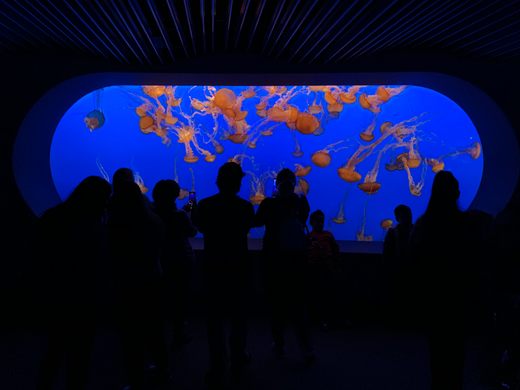The image captures a striking scene inside a commercial sea world aquarium where visitors are engrossed in viewing a mesmerizing aquatic display. Against a backdrop of deep, rich blue water, vividly colored orange and yellow jellyfish gracefully dance, highlighting the contrast significantly. The photograph, taken from behind, showcases the silhouetted outlines of approximately seven to ten people, all standing in a pitch-dark room illuminated solely by the glowing aquarium window. From behind these viewers, the contrast between the dark environment and the brightly lit window enhances the vibrant hues of the jellyfish, creating a captivating visual experience for the observers and anyone looking at the photo. The vertical, tube-shaped window adds a unique element to the scene, further emphasizing the intimacy and enchantment of watching marine life in this setting.